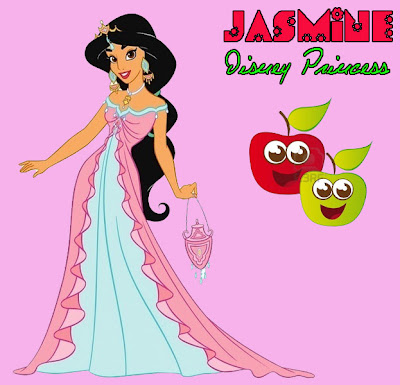This image features an illustration of Disney Princess Jasmine from the Aladdin franchise, set against a pink background. Princess Jasmine, with caramel-colored skin and long black hair, is dressed in a teal and pink outfit that includes a tiara, jade-colored earrings, and other gold adornments. She is holding a pink purse delicately in her left hand. Positioned on the left side of the image, she occupies a significant portion of the area, standing vertically.

To the right of Jasmine, and still in the middle of the image, are two apples with large googly eyes and open, smiling mouths. The larger apple is red with a green leaf, and the smaller one is green, also with a green leaf. Both apples have a playful appearance, adding a whimsical element to the image. A faint watermark with the characters "3RF" is visible on the top left of the green apple.

In the upper right-hand corner, the text "Jasmine" is written in a red, gear-adorned font with a black outline, which is somewhat unconventional for a Disney Princess theme. Below this, the words "Disney Princess" appear in a bright green script, also outlined in black. The overall style suggests an amateur mock-up of a Disney promotional design, emphasizing Princess Jasmine, the playful apples, and the untraditional text elements.